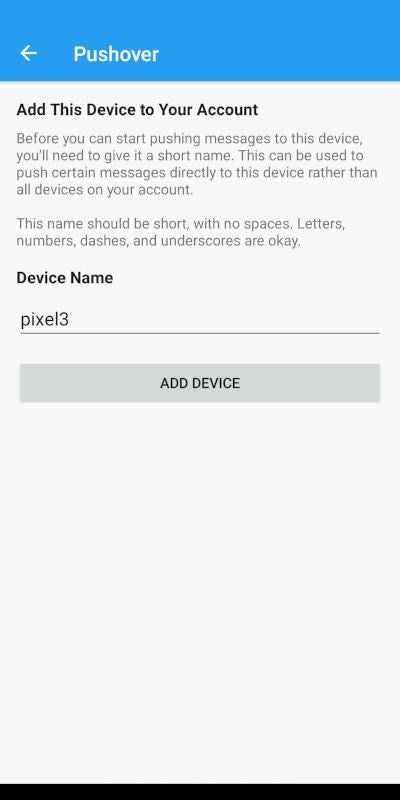The image depicts a screenshot of a mobile app interface, specifically for adding a device to an account in the Pushover app. The layout is a vertical rectangle with a whitish-gray background. At the very top, there's a prominent blue rectangular bar featuring "PUSHOVER" in a light green color and accompanied by a left-pointing arrow next to it.

Below the blue bar, a main heading in dark black letters reads "Add this device to your account." Following this, there are two paragraphs in a lighter black text providing instructions: "Before you can start pushing messages to this device, you'll need to give it a short name. This can be used to push certain messages directly to this device rather than all devices on your account. This name should be short with no spaces. Letters, numbers, dashes, and underscores are okay."

Beneath the instructions, there's a label "DEVICE NAME" also in dark black. Directly under the label is a long black input bar where the user has entered the device name as "PIXEL3."

Further down, there's a long, gray rectangular button labeled "Add Device." At the very bottom of the image, a black bar spans across the width, completing the interface.

Overall, the screenshot illustrates the process of adding a device named "PIXEL3" to a Pushover account, highlighting key visual elements and user input areas.